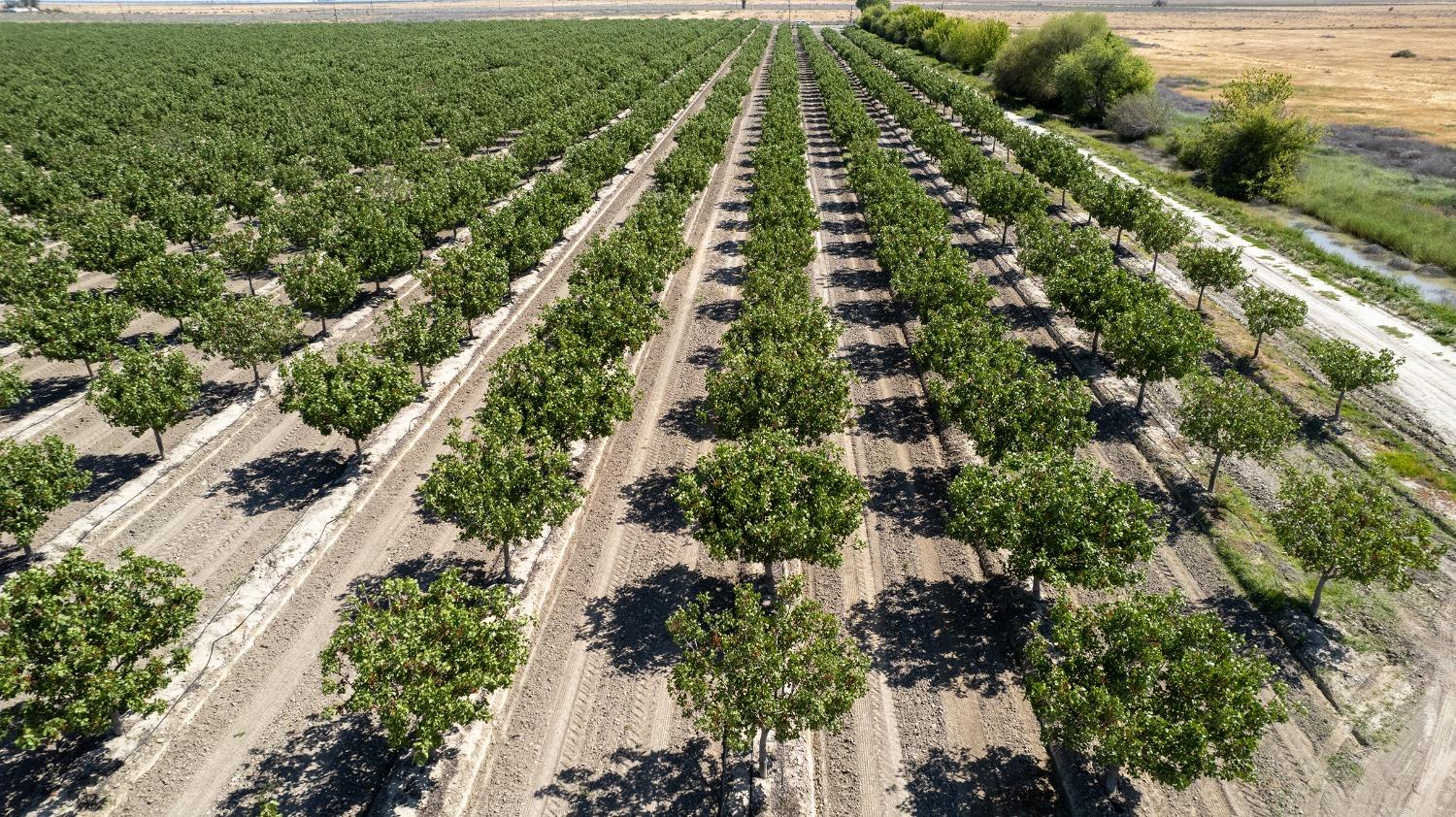The aerial photograph captures an extensive tree orchard stretching hundreds of yards into the distance. The meticulously planted trees form distinctive, even rows, with each tree being remarkably similar in size, shape, and color. The trees, which lack fruit, have thin trunks adorned with leaves predominantly at the tops. The light brown dirt paths between the rows are flattened and marked with tire tracks, designed for vehicle access and irrigation. Shadows cast by the sunlight on the right-hand side fall on the left, highlighting the spacing and symmetry. To the right of the orchard, a line of low-lying brush and trees leads to a golden field that transitions into shades of purple and green. A small canal, filled with rainwater, and a dirt road further define the boundaries of the orchard. In the lower left-hand corner of the photograph, a small structure and cars are visible, adding context and scale to the expansive, serene landscape.